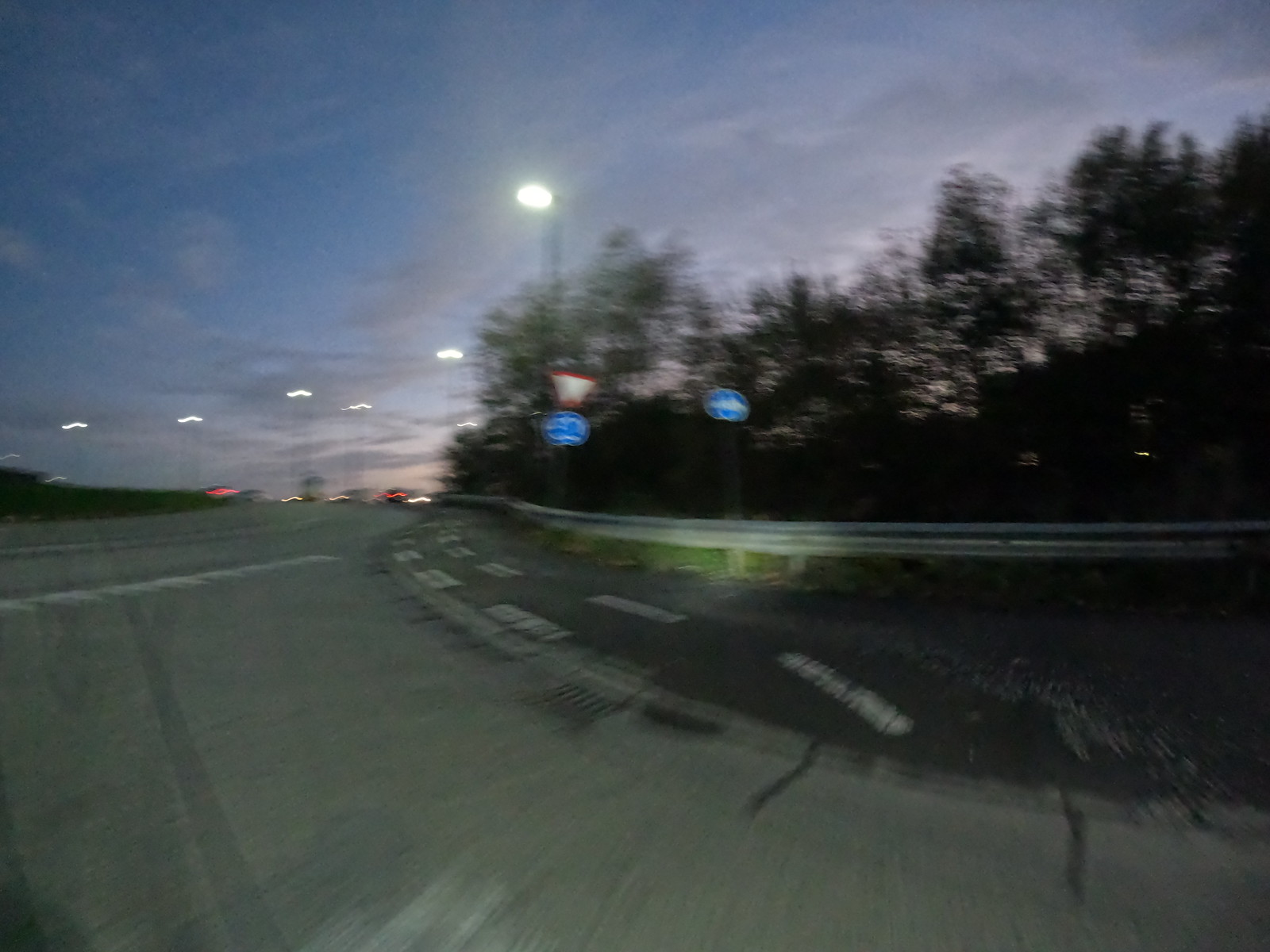The image is out of focus, depicting what appears to be a roadway, potentially an on-ramp, with several distinctive elements. From the center stretching to the right side, there is a visible guide rail. Two bluish round signs are prominently displayed, one of which features a red triangle overlaying a white interior. The roadside is lined with multiple pole lights. On the right side of the frame, various trees are scattered, blending towards the center. The left side of the image shows a patch of green, possibly grass, suggesting this area is on the opposite side of the road. The sky at the horizon transitions from light blue to a light tan or light red hue, hinting at either sunrise or sunset. There is a faint glare of headlights reflecting off the guide rail, adding a subtle brightness to the scene.